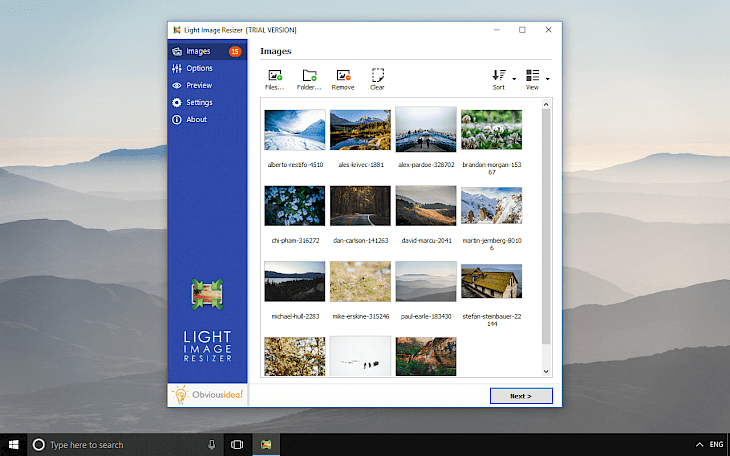The image depicts a software interface, specifically the Light Image Resizer trial version. The background is adorned with an array of gentle, rolling mountains shrouded in fog, offering a serene and misty landscape. In the foreground, a prominent dialog box outlines various functionalities of the software. The top section of the box features options such as "Images," "Folder," "Remove," "Clear," "Sort," and "View."

Within the dialog box, there are 15 images arranged in a grid layout – three rows consisting of four images each, and a final row with three images. Each image has text beneath it, though the text is too small and blurred to be legible. 

On the left side of the interface, a blue sidebar presents further options, listed from top to bottom: "Images" accompanied by an orange circle with the number 15, "Options," "Preview," "Settings," and "About." At the bottom of this section, there is a depiction of a box with three green arrows converging at its center, alongside the text "Light Image Resizer." In the lower right corner of the dialog box, a gray button labeled "Next" is visible, ready to guide the user to the subsequent step in the process.